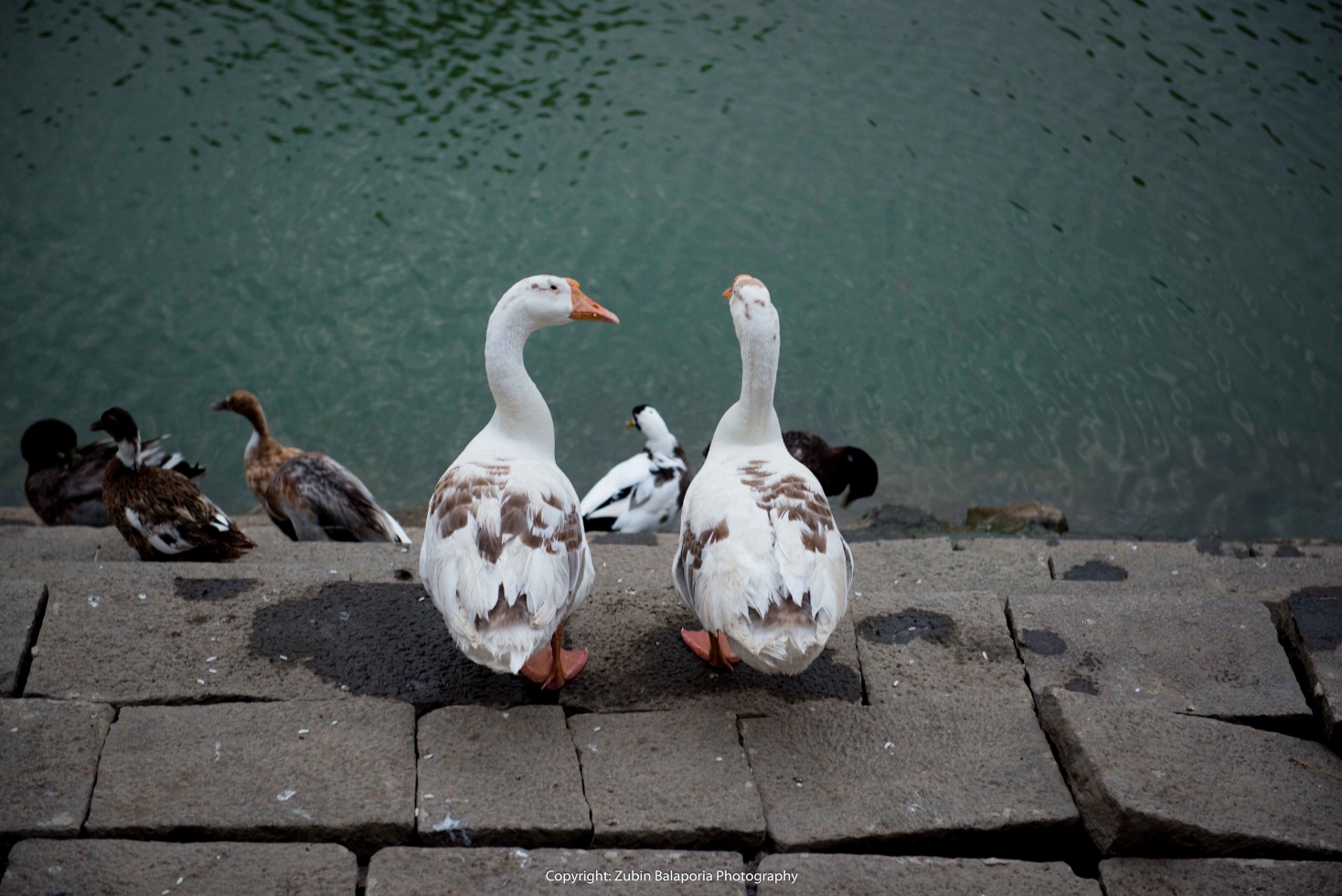This image captures seven ducks perched on uneven, aging concrete steps that descend into a dark green, man-made lake. Dominating the foreground, two white ducks with scattered brown feathers, orange beaks, and orange feet stand with their backs to the camera. Below them, a third white duck with black and white spotting is closer to the water. In the background, on the left side of the steps, four more ducks with darker plumage in shades of brown, black, and gray add contrast to the scene. The disorganized, cinder block-like steps occupy the lower half of the image, while the serene lake envelops the upper half. Notably, the image bears a copyright mark from Zubin Rapolor Photography at the bottom center.